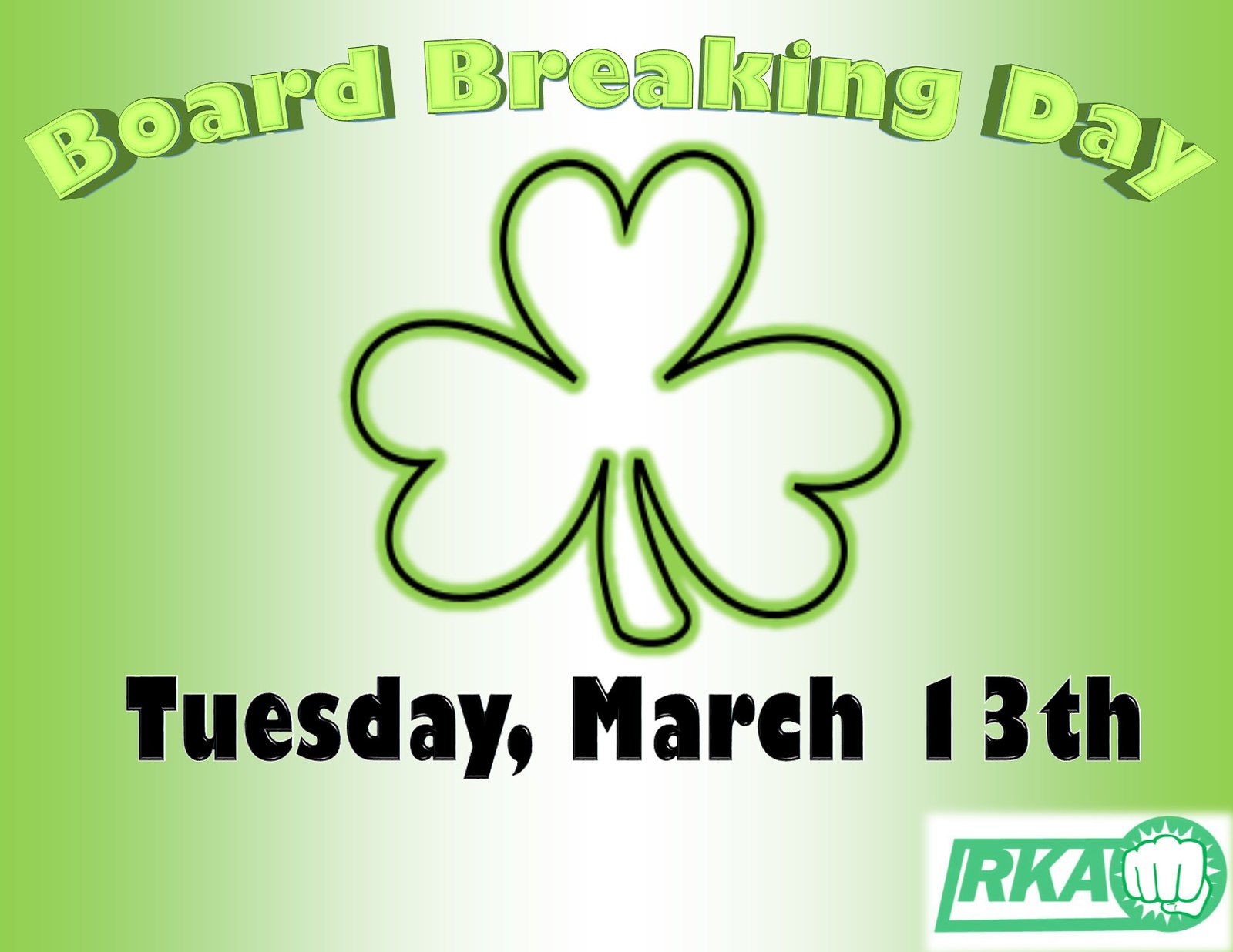The image showcases a promotional sign for an event. The background features a gradient that transitions from lime green on the edges to a bright white in the middle, and back to lime green. At the top, in chunky, light neon green font with a shadow effect, it reads "Board Breaking Day." Below this title, there is an outlined three-leaf shamrock, bordered in neon green and black. The event's date, "Tuesday, March 13th," is prominently displayed in black font beneath the shamrock. In the lower right corner, the sign features a small white rectangle that contains the letters "R.K.A." to the left of a circle with a fist inside it. The overall aesthetic of the sign suggests an Irish theme, but the specifics of "Board Breaking Day" remain unclear.